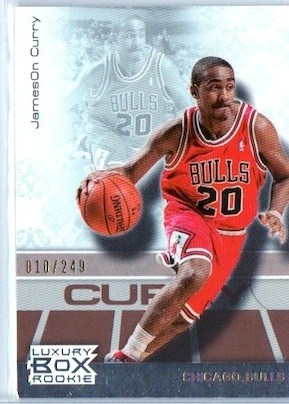This portrait-oriented close-up image of a collectible sports card features Chicago Bulls player Jameson Curry. Positioned on the right side, Curry, an African-American man with very short black hair, is captured in motion, dribbling a basketball with a serious look of concentration on his face. He wears a red Bulls jersey with "BULLS" and the number 20 in black lettering, along with a visible white sock. The card's background includes a faded, black-and-white version of the same image, creating a layered effect. Along the left side, in vertical black text, the name "Jameson Curry" is inscribed, with a capitalized "O" in Jameson. At the bottom, golden embossed text reads "010/249," indicating this specific card is number 010 out of a 249 limited edition series. Partially obstructed text in maroon appears below, possibly spelling "CURRY." The bottom left corner features a logo with "Luxury Box Rookie," while a strip along the bottom right reads "Chicago Bulls" in a combination of representational photography and graphic design.